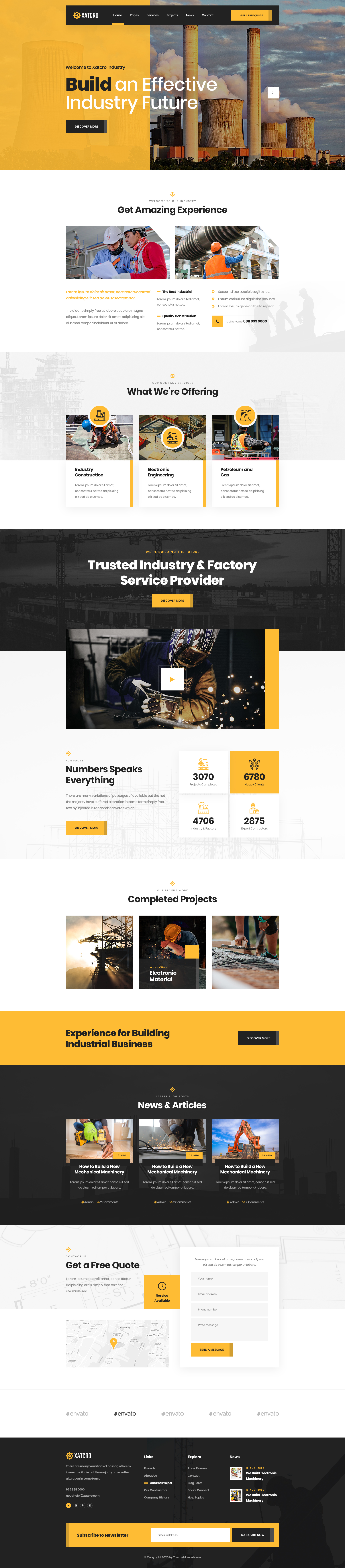The image is a detailed screenshot of a multi-section webpage belonging to a business named "XATCRO". At the top of the page, the header features the tagline "Build an Effective Industry Future" against a backdrop depicting a factory with large towers emitting smoke, emphasizing the industrial focus of the company. The color scheme throughout the webpage includes notable contrasts of black and a shallow orange.

As the webpage content is explored from top to bottom, several key sections are highlighted:

1. **Header**: Displays the company name "XATCRO" and the tagline.
2. **Section 1**: Promotes the message "Get Amazing Experience" followed by "What We're Offering".
3. **Section 2**: A statement reads "Trusted Industry and Factory Service Provider".
4. **Section 3**: Features the phrase "Numbers Speaks Everything", accompanied by a box displaying various numerical metrics, although the text is too small to decipher.
5. **Section 4**: Highlights key offerings with "Completed Projects" and "Experience for Building Industrial Business".
6. **Call to Action**: Encourages visitors to "Get a Free Quote".
7. **Footer**: Presents a black rectangle containing additional information, keeping with the design theme.

The webpage layout is structured to guide the viewer through the company's services, achievements, and contact actions effectively, with a strong visual emphasis on the industrial sector.